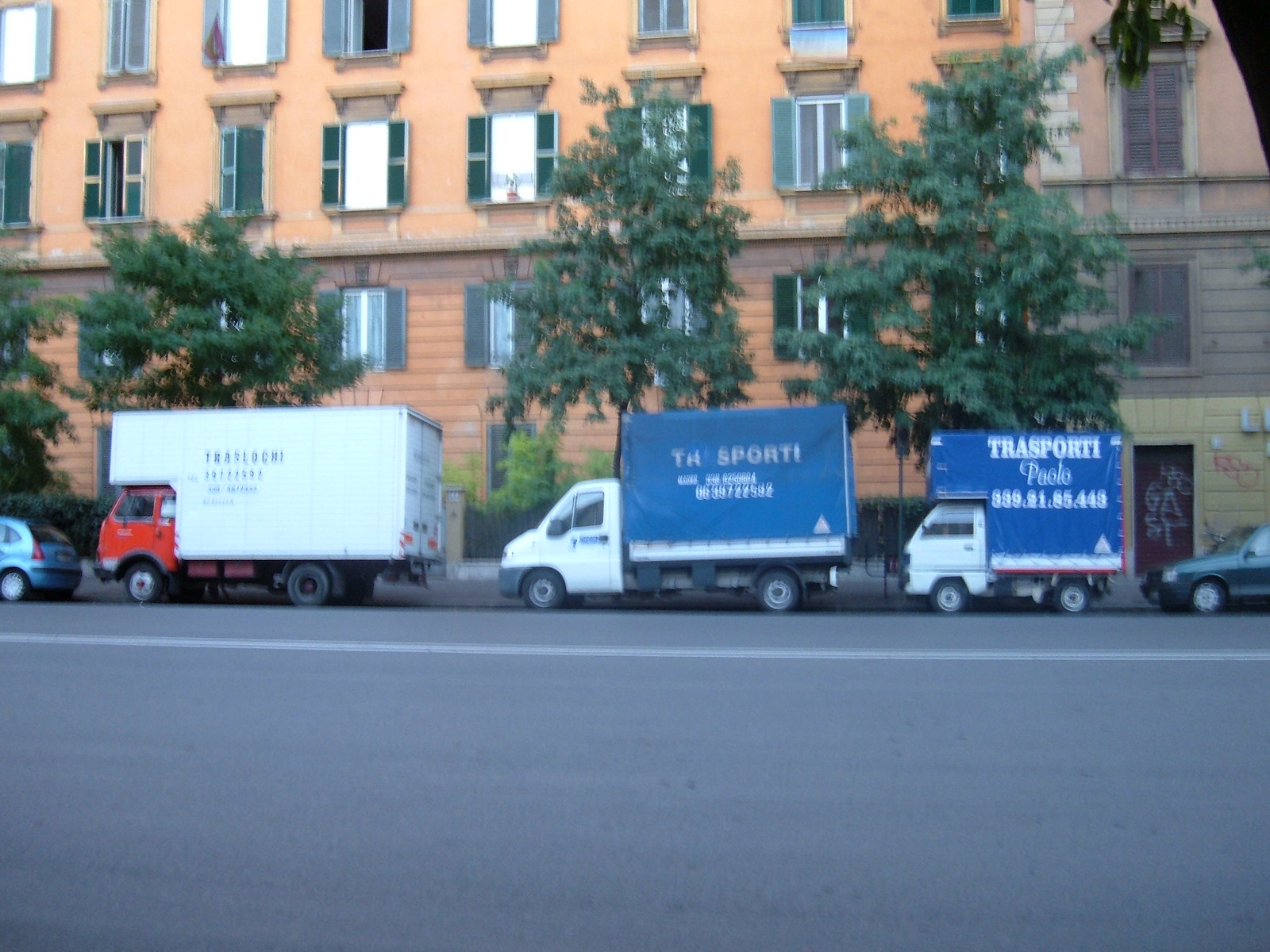The photograph captures a slightly blurry scene taken from across a road with a white line marker, featuring an apartment building in the background. The building is peach-colored with noticeable graffiti on its door and flanked by four green trees and several bushes behind a gate. In front of the building, there are five parked vehicles: prominently three trucks varying in size, and two smaller vehicles partially in frame on either side. 

The largest truck, positioned on the left, has a red cab and a white trailer with some indistinct writing. The second truck, slightly smaller, has a white cab and a blue trailer marked "TH Sport" along with a barely legible phone number. The smallest is a "baby" truck with a white cab and a blue trailer that reads "Tri Sporty Palo," though the accompanying phone number is also unclear.

Completing the row of vehicles, a blue car is parked in front of the first truck, and another smaller car can be seen behind the last truck.